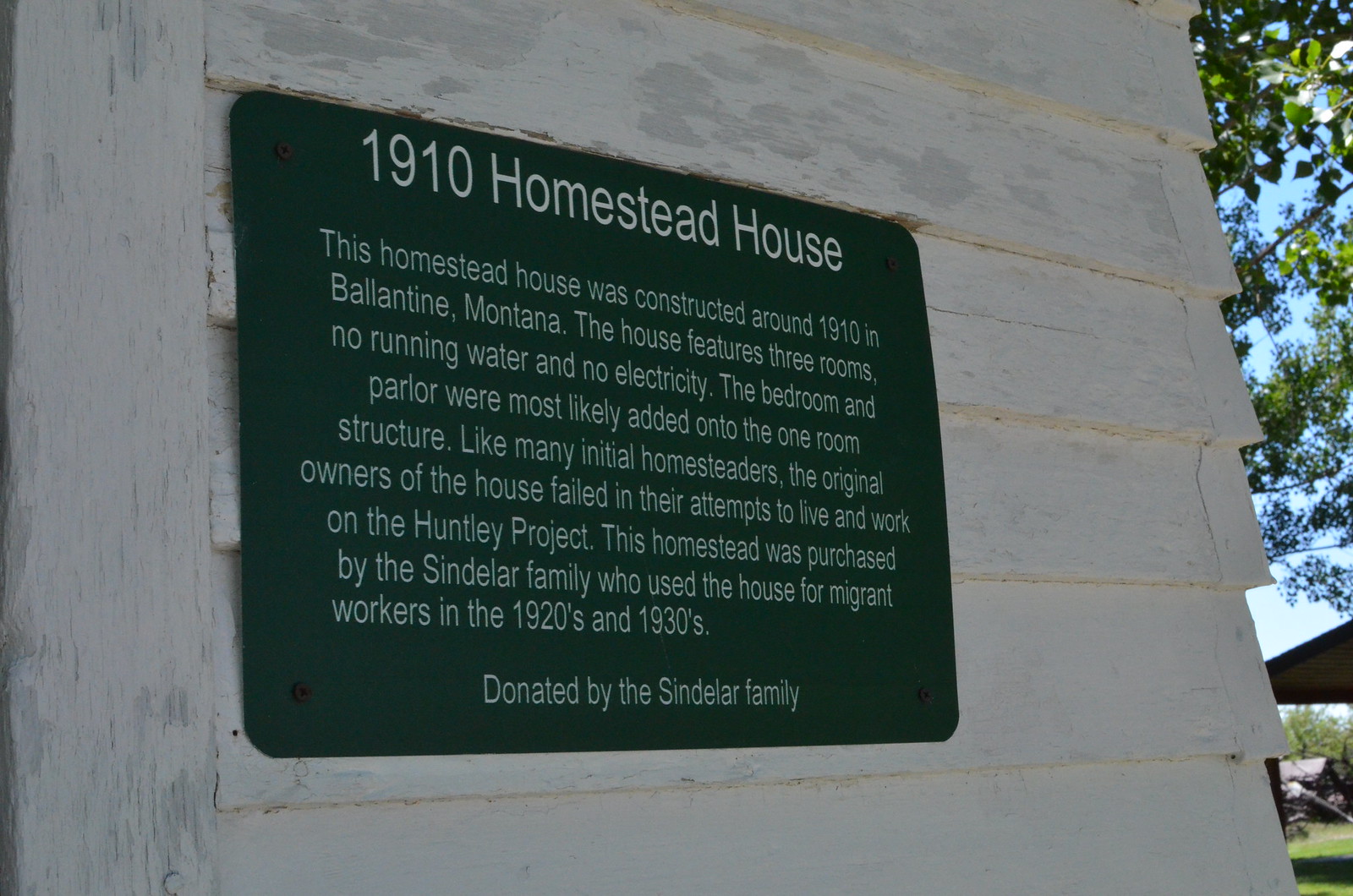The image depicts the side of a historic wooden building, painted white with horizontal slats that exhibit signs of wear but remain in fair condition. Prominently featured in the center of the image is a black plaque with white lettering. The plaque reads "1910 Homestead House" in large text across the top. Below it, in smaller text, it provides historical context: "This homestead house was constructed around 1910 in Ballantyne, Montana. The house features three rooms, no running water, and no electricity. The bedroom and parlor were most likely added on to the original one-room structure. Like many initial homesteaders, the original owners of the house failed in their attempts to live and work on the Huntley Project. The homestead was purchased by the Sindler family, who used the house for migrant workers in the 1920s and 1930s. Donated by the Sindler family." Surrounding the building, you can see patches of grass, a blue sky, and trees, indicating that the setting is outdoors on what appears to be a clear day. The colors present in the scene include shades of white, gray, green, tan, blue, and brown.